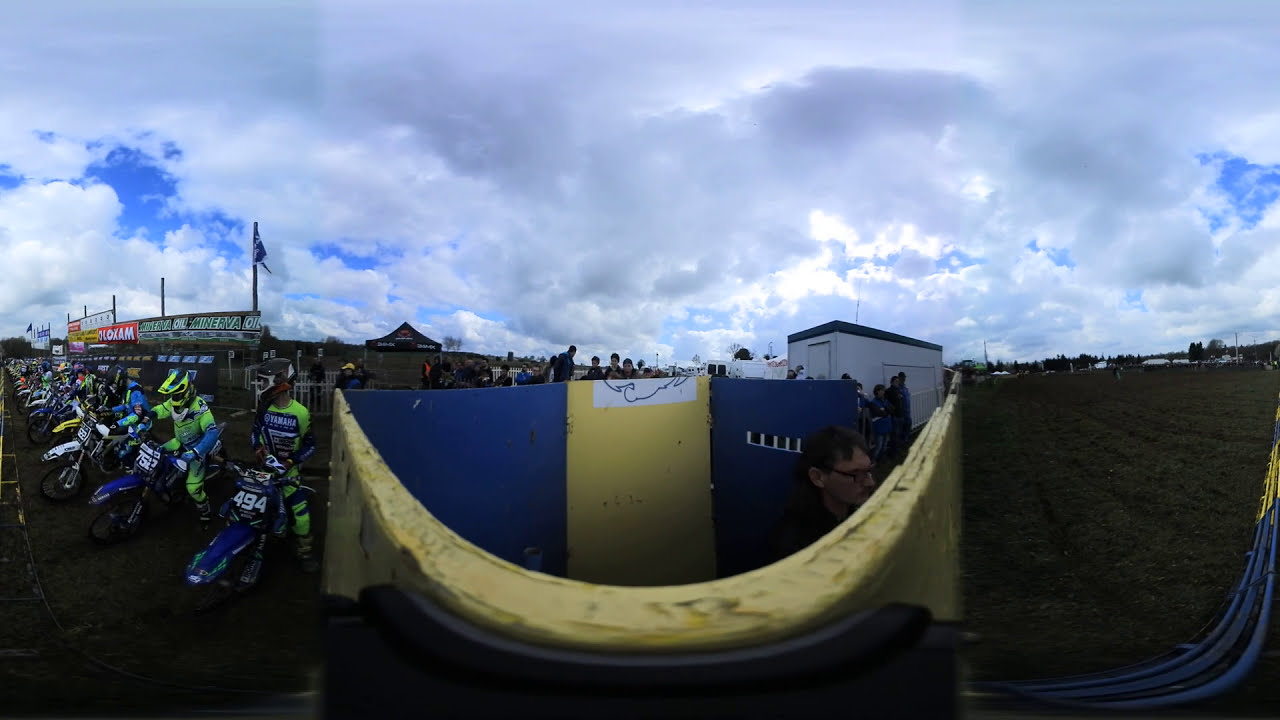The photograph captures the electrifying moment just before the start of a motorcycle race, viewed through a fish-eye lens that adds a unique, slightly distorted perspective to the scene. On the left, a row of motorcyclists on blue, white, and yellow bikes sit poised at the starting line, clad in full protective gear including pants, jerseys, gloves, and helmets. Behind them, a stadium adorned with various sponsorship banners and flags looms large. In the center of the image, a man wearing spectacles stands inside a blue and yellow booth-like structure. To the right, a yellow horseshoe-shaped barrier and a white-and-yellow wall define a pit area, with spectators above looking down. Beyond this, a small white building is visible, set against an open field of grass. The sky overhead is densely packed with fluffy white clouds that occasionally part to reveal patches of blue and a hint of sunlight, adding a dramatic backdrop to the charged atmosphere at the race starting line.